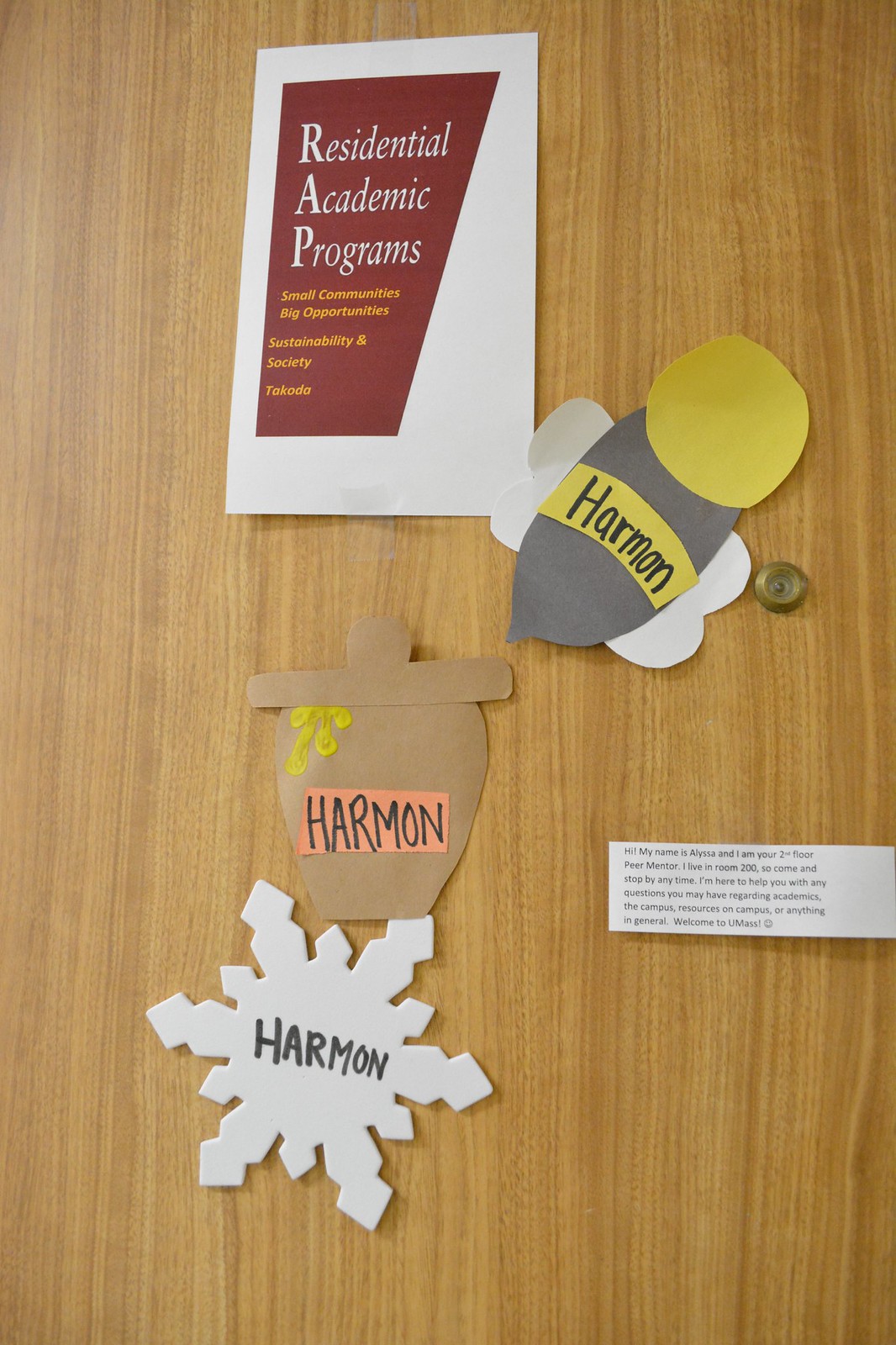This image features a brown wooden door adorned with several decorative and informational elements. Central to the display is a maroon and white piece of paper taped to the door, titled "Residential Academic Programs” in bold white text. The document highlights themes of "Small Communities, Big Opportunities, Sustainability, and Society," with the word "Dakota" printed in yellow at the bottom. 

Adjacent to this is a creatively crafted bumblebee, made from construction paper in shades of gray, yellow, and white, prominently labeled "Harmon." Below the bee, there is a handmade brown flower pot, also marked with the name "Harmon." A little further down hangs a white paper snowflake, similarly inscribed with "Harmon."

Additionally, a smaller white piece of paper mentions a welcome message from someone named Alyssa, who identifies herself as the second-floor peer mentor living in room 200. The text encourages residents to visit her for help with any questions. The arrangement appears to serve as a welcoming display for new residents at UMass, blending practical information with creative, personalized decorations.